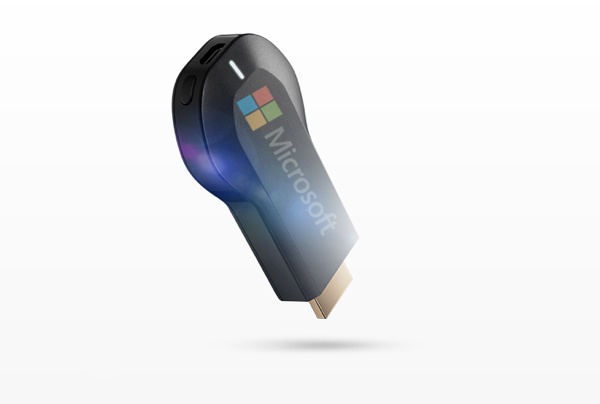The image features a black, rectangular USB thumb drive with a rounded end, positioned against an all-white background with a small grayish shadow beneath it. The USB connector is visible at the squared end with no protective cap. The drive prominently displays the word "Microsoft" in slightly washed-out color towards the bottom, and below the text is the iconic four-colored Microsoft logo, consisting of red, blue, yellow, and green squares forming a larger square. A narrow white vertical line is located near the rounded edge of the device. The overall orientation of the thumb drive is nearly vertical, tilted slightly to the left. The device's surface is reflective and metallic, adding to its sleek appearance.